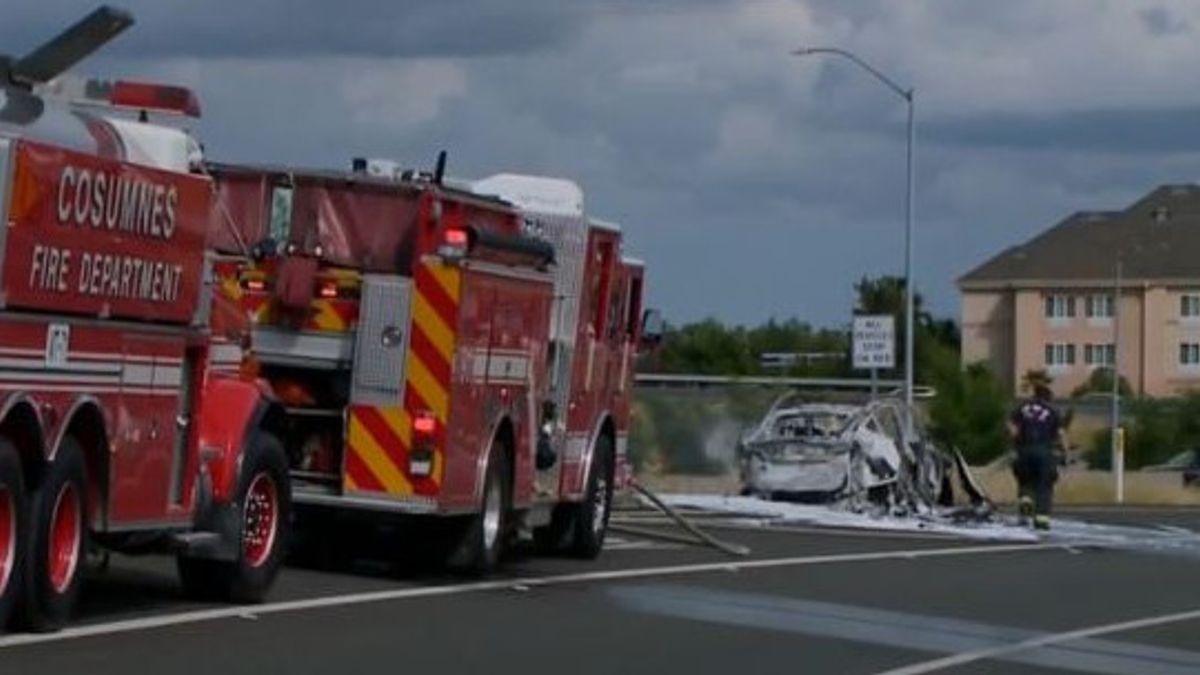This is a color photograph captured on a dark, cloudy day depicting the aftermath of a severe car accident. Dominating the middle-right of the image is a white, sedan-like car, utterly destroyed and charred, likely from a fire. The car, now an ashen shell, sits near a light post and a black-and-white sign, which is unreadable due to the image’s focus. Behind the car, a significant amount of water is visible, probably discharged while extinguishing the flames.

Adjacent to the car, on the left side, are two fire trucks, painted in red with yellow and red stripes, bearing the inscription "Cosumnes Fire Department," indicating a location in California. One fire truck reveals a tiny part of its front right door and the rear, while the other displays its side and front right tire. A firefighter is seen on the scene, walking towards the car, suggesting active emergency response.

In the background, towards the right, lies a multi-story building, possibly a hotel or a residential structure, showcased with light-colored bricks and a brown roof. Adding to the detailed setting are the observable cloudy and overcast skies, enhancing the somber mood of this tragic scene. The whole event unfolds on a parking lot or a street lined with asphalt, evoking a sense of a typical residential or commercial area amidst an unexpected calamity.